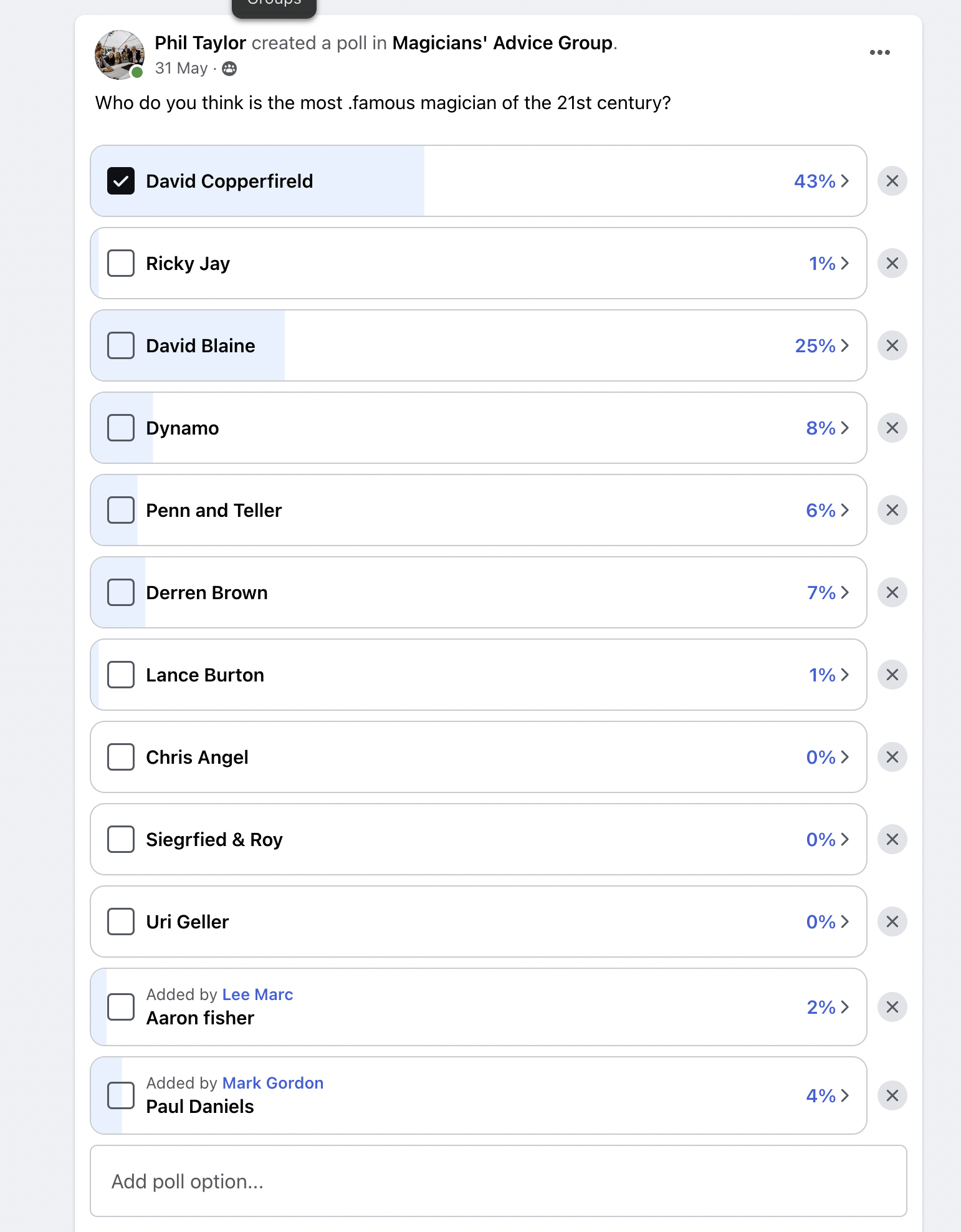This detailed screenshot from a smartphone captures a poll created by Phil Taylor in the Magician's Advice Group, presumably on a social networking site with a predominantly white background and light blue borders on either side. Although the platform is unspecified, it is suggestively from a Facebook group.

In the upper-left corner, Phil Taylor's name and an indistinct profile photo—potentially depicting a forest under a gray sky—are visible. The poll, dated May 31st, inquires, "What do you think is the most famous magician of the 21st century?" The poll results are displayed below the question.

David Copperfield leads the poll with 43% of the votes, indicated by a black square with a white checkmark beside his name. The subsequent magicians and their respective vote percentages are listed as follows:
- Ricky Jay: 1%
- David Blaine: 25%
- Dynamo: 8%
- Penn and Teller: 6%
- Derren Brown: 7%
- Lance Burton: 1%
- Criss Angel: 0%
- Siegfried and Roy: 0%
- Uri Geller: 0%
- Aaron Fisher: 2%
- Paul Daniels: 4%

This poll showcases the diverse opinions within the magician's community regarding the most renowned magician of the current century.